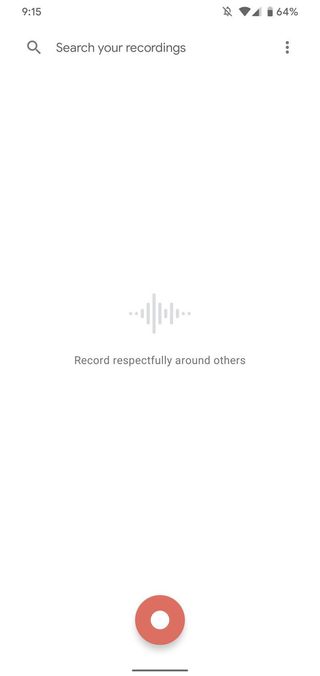The image depicts the screen of a user's cell phone with a white background. At the top-left corner of the screen, the time is displayed as "9:15 AM" in black text. On the top-right corner, there is an icon showing the battery life at 64%, alongside indicators for notifications and a silenced phone, with three bars of signal strength visible.

Below this top section, on the left-hand side, there is a black magnifying glass icon, followed by the phrase "Search your recordings" in black text. On the far right, three vertical dots are displayed as a menu icon.

The screen has substantial white space until about halfway down, where a message in gray text reads, "Record respectfully around others." Beneath this message, there are sound file lines representing audio activity, consisting of alternating longer and shorter lines.

Further down, additional white space leads to a red circular button at the bottom-center of the screen. This button features a small white circle in its center and has a very short, thin black line directly underneath it, indicating the recording function.